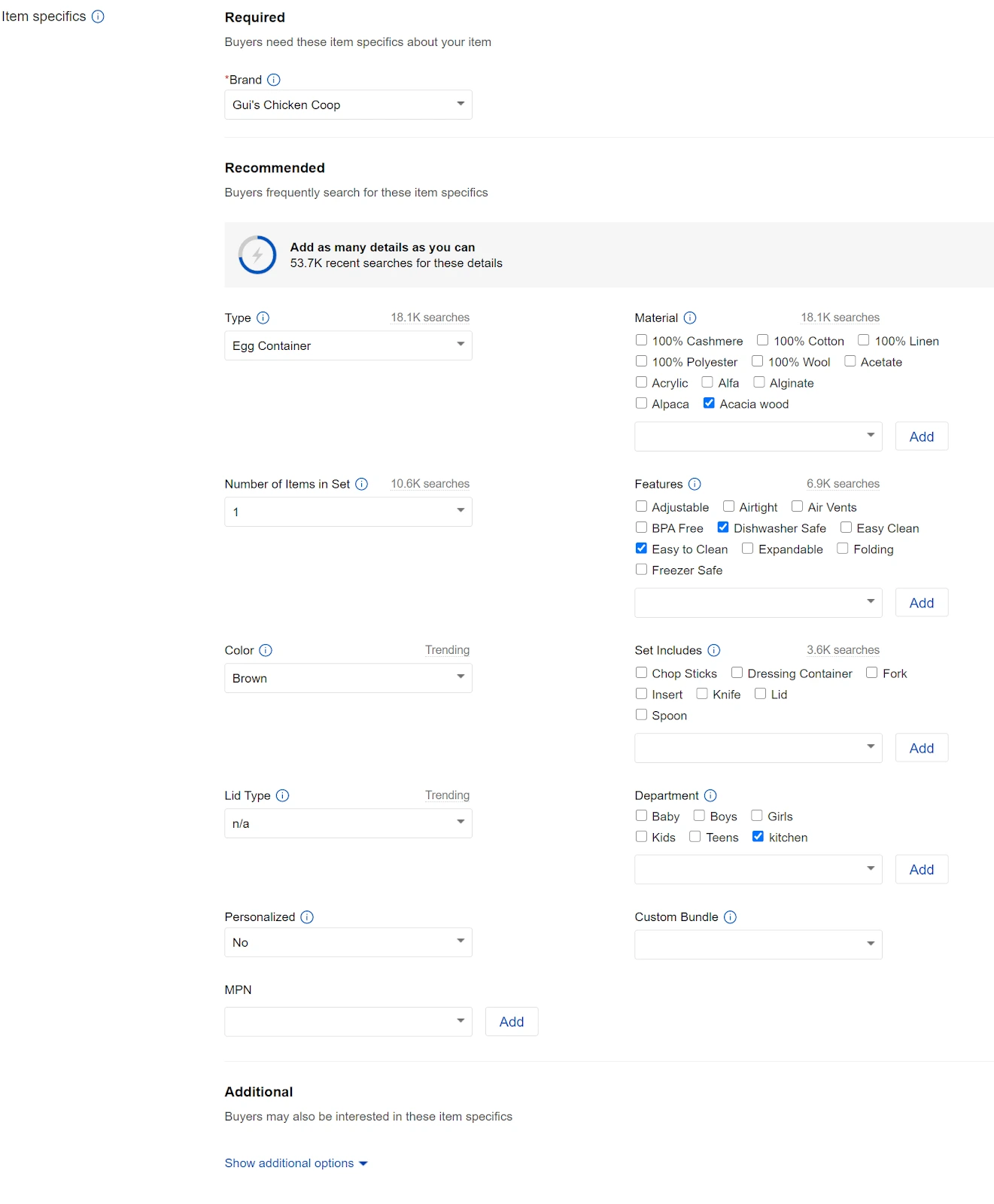**Detailed Caption:**

A detailed screenshot of a section of a product listing webpage on a website with a clean, white background. The page emphasizes the importance of providing specific item details for the benefit of the buyers. At the top, there's a highlighted notice indicating the required specifics for items, which are marked as particularly important for better search results and buyer visibility.

In the middle of the screenshot, there's an icon featuring a predominantly blue circle with a gray segment on one side and a thunderbolt symbol in the center, signifying high priority or attention.

Beneath this, there is a comprehensive list with clear labels and values for various product attributes:
- **Brand:** Required
- **Type:** Egg Container (or similar with a starting 'C')
- **Material:** (Not specified)
- **Number of Items in Set:** 1
- **Features:** Dishwasher Safe, Easy to Clean
- **Color:** Brown
- **Lid Type:** Not Applicable (noted as N/A)

Each of these attributes is laid out in a structured list format, making it easy for the user to input and review the necessary details for the product listing.